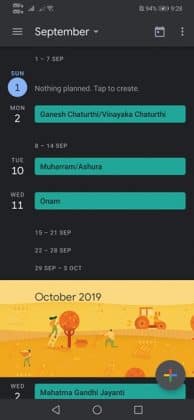In this image, we have a black background featuring a detailed calendar layout. Starting at the top, there are three small lines next to the word "September", followed by a small white icon. Below this, a calendar is displayed with three dots representing options or settings and "Sunday the 1st" encircled with the words "nothing planned, tap to create."

Following the start of September, the calendar specifies:
- Monday, the 2nd.
- A green box highlighting "Ganesh Chaturthi" and "Vinayaka Chaturthi."
- A weekly overview from the 8th to the 14th of September, with "Tuesday the 10th" marked in a green box for "Muharram/Ashura."
- "Wednesday the 11th" also highlighted for "Onam."

Further, the calendar displays the segments of September:
- The 15th through the 21st.
- The 22nd through the 28th.
- And the 29th of September through the 5th of October.

Beneath the September calendar is an image labeled "October 2019" with autumnal colors—yellow and orange—and a scene depicting pumpkins and people working on a farm. Prominently featured is a large dark circle with a multi-colored plus sign (in red, yellow, blue, and green).

The bottom section highlights:
- "Wednesday the 7th" in a green box with the note "Mahatma Gandhi Jayanti."
- Symbols for navigation or options, including a triangle, a circle, and a square.

This comprehensive visual representation provides a clear and organized view of upcoming events and dates for September and early October.